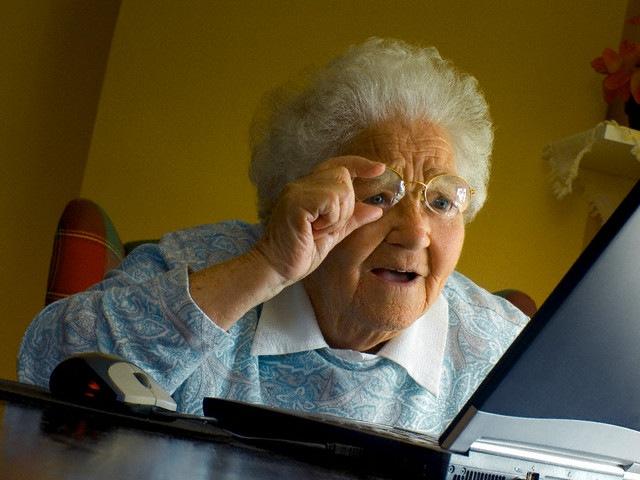The image features an elderly woman with short, white, puffed-up hair typical of older generations, and a face marked by numerous wrinkles. She is of Caucasian descent and is seated in a chair with a partially visible plaid pattern in green and red, situated in a room painted a darker shade of yellow. 

In the top right corner of the image, there is a decorative white shelf that holds some objects, though they aren't clearly discernible. The viewpoint of the image is slightly slanted, providing a unique perspective.

The elderly woman is holding up a pair of circular, gold-rimmed glasses with a surprised and confused expression, as if questioning the reality of what she is seeing. She is dressed in a blue and white sweater adorned with a swirling pattern, beneath which she wears a white collared shirt.

In front of her is a laptop with a blue and navy blue lid and a gray base. The laptop is plugged in, with a black cord extending off the table. Alongside the laptop, there is a mouse that has a white scroll wheel, a dark blue body, and a red light indicating it is in use.